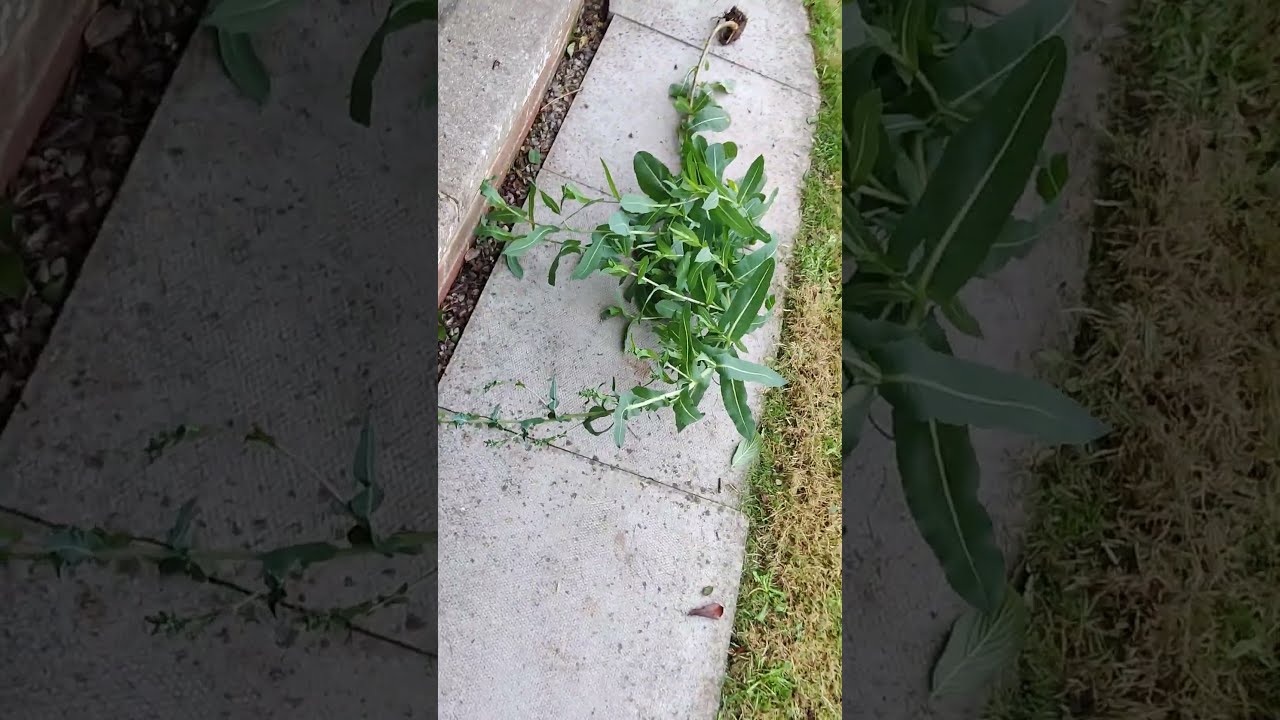The image consists of a three-frame composition with the main central frame depicting a top-down view of a small pile of greens or weeds on a concrete or brick surface. The weeds, seemingly not growing but rather placed or thrown there, rest atop the slab, with their reluctant appearance accentuated by the juxtaposition. Adjacent to this area is a patch of grass, partially brown and partially green, indicative of a lawn that appears poorly maintained. The sidewalk or paved area surrounding the central scene is formed by large, square slabs, approximately 12x12 inches, with a narrow gravel-filled separation between the slabs and the sidewalk.

The side frames on the left and right are magnified and underexposed sections of the main image, rendering them dark and difficult to discern, focusing close up on the left and right parts of the weed pile without revealing the broader context supplied by the central frame. The overall tint and magnification in the side frames obscure finer details, reinforcing the importance of the primary, brightly-lit central frame. The rectangular image's surroundings show an edge and gap between the pavers, lacking substantial context to identify the specific location.